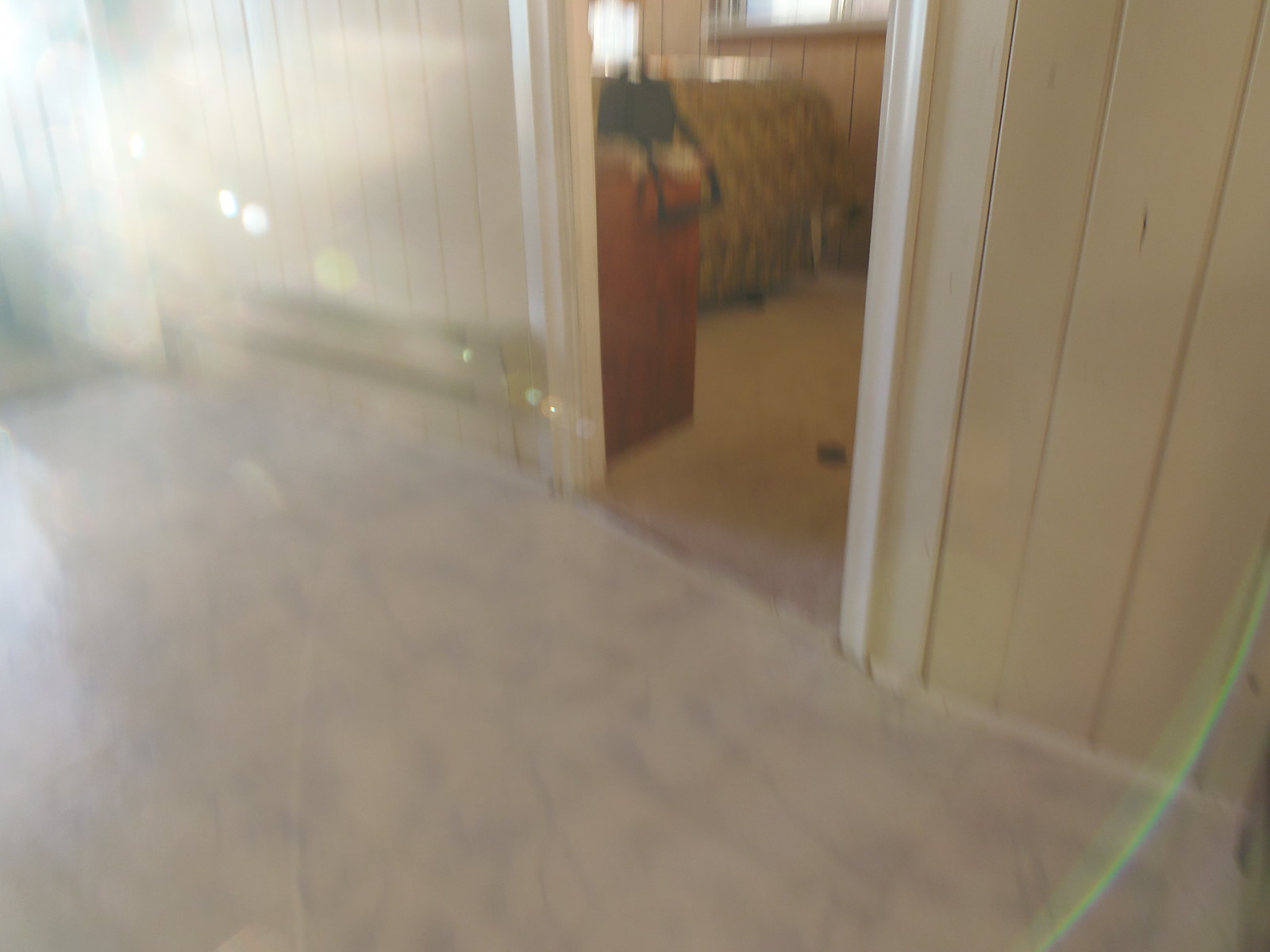This photo, taken indoors and characterized by its blur, showcases a room with distinct paneling and sunlight effects. The walls and the woodwork surrounding the space are painted a light cream color, accented by a white-trimmed doorway located almost centrally in the upper part of the image. This doorway leads into another room, further enhancing the depth of the picture.

The carpet in the immediate foreground appears to be a tan or cream color, reflecting sunlight, which conspicuously floods the upper left portion of the photo with a bright white glare. This sunlight, likely coming from an off-camera window, results in small white and yellowish reflective spots in the upper left and a subtle rainbow effect, predominantly green and purple, in the lower right corner.

Inside this secondary room, partially visible through the doorway, are a few discernible items despite the blurriness. A possible dark wood dresser and the back of a couch, which may be green in color, are set against the far wall. Atop this dresser, there appears to be a black purse or bag, adding a touch of detail to the composition. Overall, the image captures a quiet interior scene, enhanced by natural light and household furnishings amidst the blur.